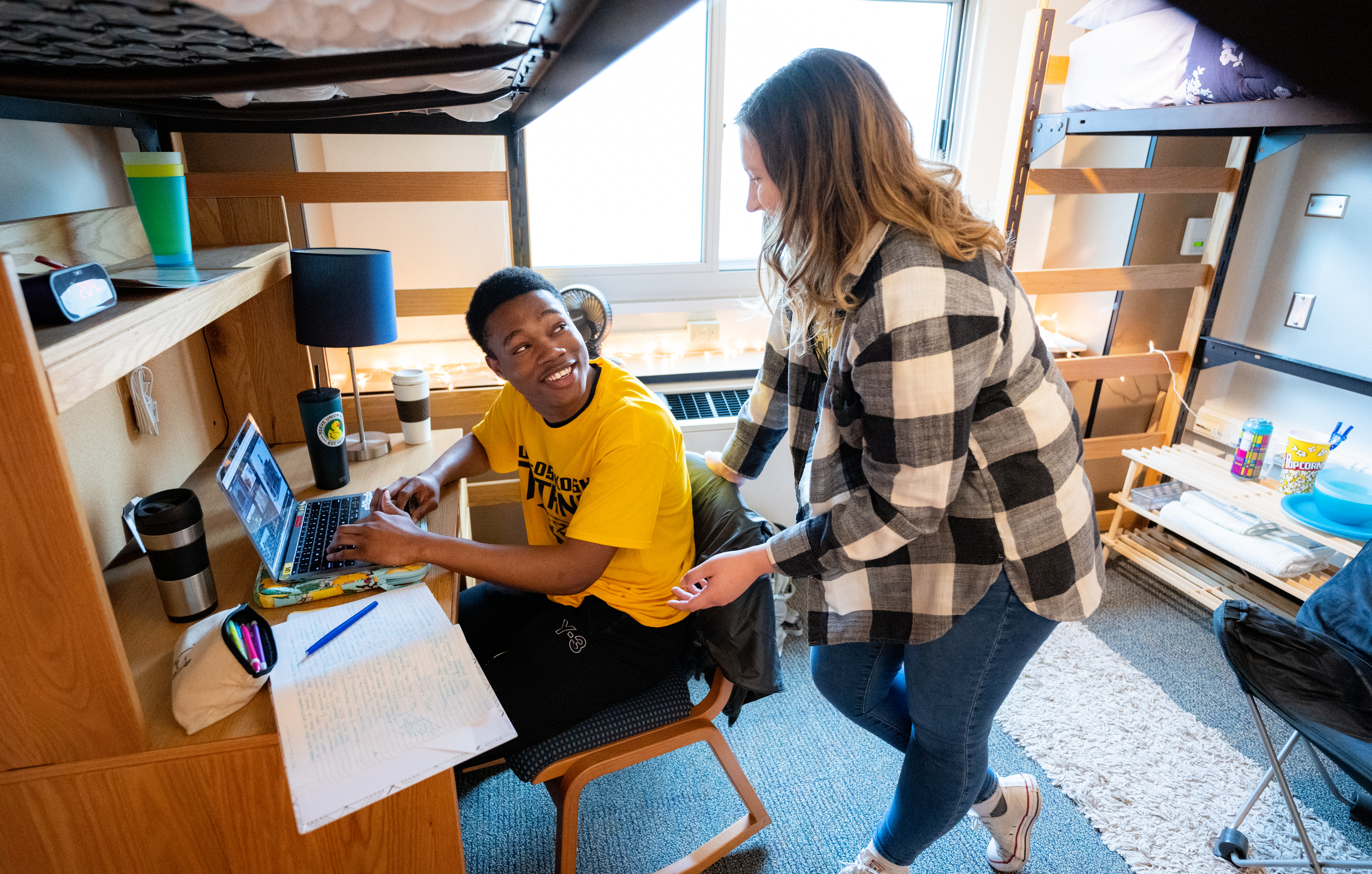In the photograph, two people are situated within what appears to be either a bedroom or a dorm room. The room is centered around a window with two large panes of glass, separated by a gray sill and framing, allowing sunlight to flood the scene. In the foreground, the young man, wearing a yellow T-shirt with black writing and black pants, is seated at a brown desk, with his legs tucked under it. He is turned slightly to the left, looking back at the woman standing behind him. His desk is cluttered with various items: an open laptop perched on a protective case, a reusable mug, a cup, a pad of paper with a blue pencil atop, a bag filled with pencils, an alarm clock, and a lamp with a blue shade.

The woman, who stands leaning slightly against the back of the chair, has long brown hair cascading past her shoulders. She is dressed in a black, white, and gray checkerboard jacket, blue jeans, and white tennis shoes. Her right hand rests on the chair back, and her left hand extends in front of her. They appear to be engaged in conversation, with the young man smiling as he looks at her.

The background reveals more details of the room: closer to the window, a radiator sits on the floor. To both the left and right of the image, wooden ladders with brown steps hint at bunk beds, with the top bunk visible in the upper right corner and the underside of another bed in the upper left. Additionally, behind the subjects, a table can be seen bearing cups, bowls, and plates, adding to the room's lived-in ambiance.